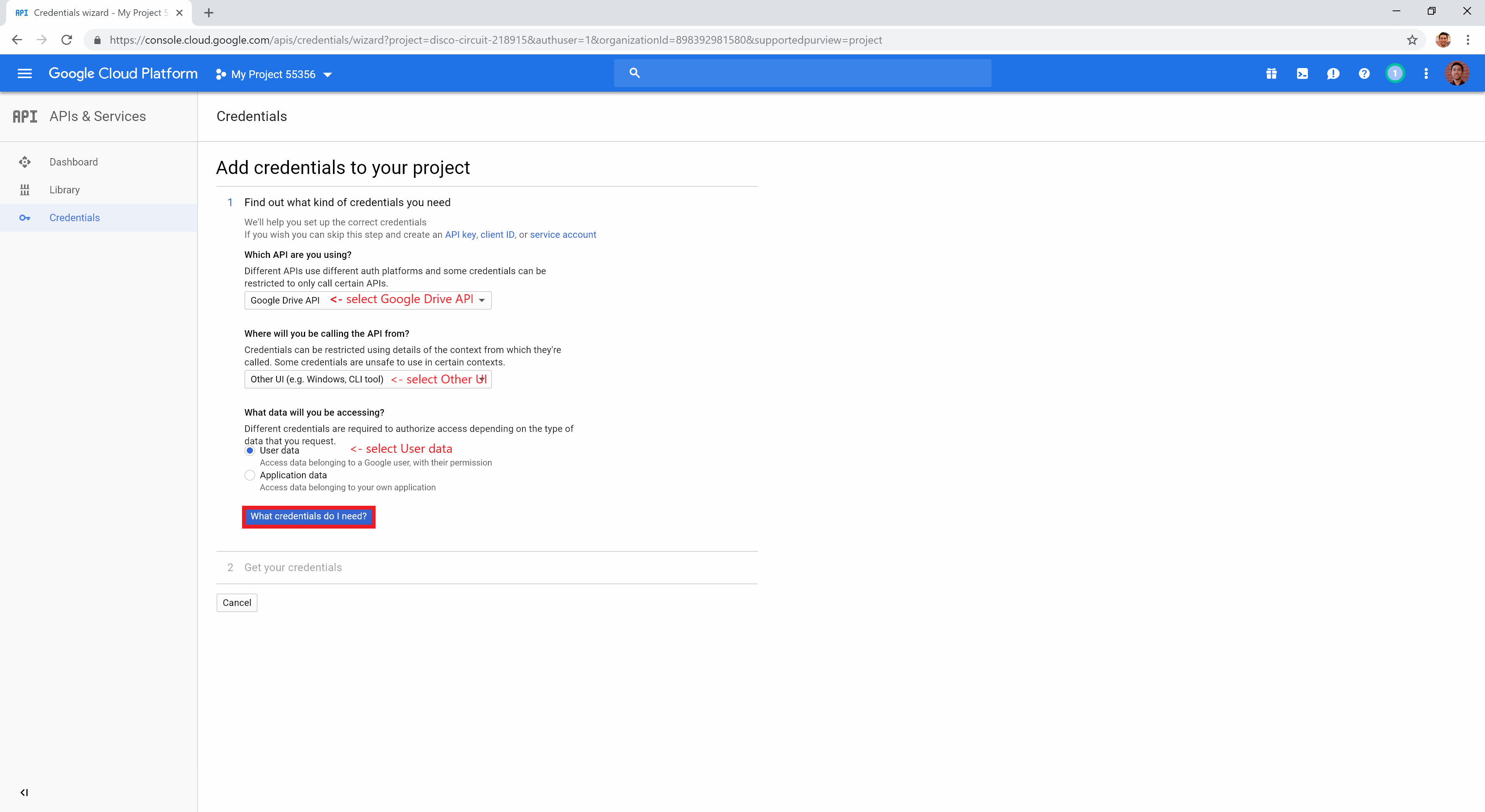The image displays a detailed interface of the Google Cloud Platform's web console. At the top is a gray search bar, followed by a light gray search bar with the faint text "console.cloud.google.com" inside. Below this section is a blue text bar stating "Google Cloud Platform," adjacent to which are the words "My project" and a white arrow pointing downwards. 

Underneath, there is the heading "Credentials," with the left side showing the uppercase label "API" and beside it, "APIs and Services." To the right, there is a prompt saying "Add Credentials to Your Project," followed by a series of steps:

1. "Find out what kind of credentials you need."
2. "What API are you using?" This line includes a clickable red text option labeled "Select Google Drive API."

Next, there is another clickable area in black text asking, "When will you be calling an API trust?" which is followed by, "Your data is accessing." Below this, in red text, is a clickable option labeled "Select user data," with an arrow pointing to the left.

Finally, at the bottom of the image, there is a blue rectangle outlined in red, containing small white text inside.